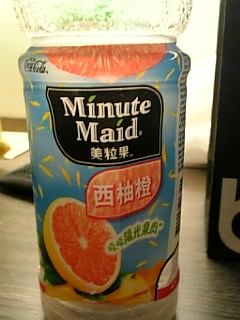The image is a clear, color photograph of a plastic container of Minute Maid grapefruit juice. The container features a sky blue label with a black square at the top, where "Minute Maid" is written in white font. Both "I"s in "Minute" and "Maid" are dotted with green leaves. The label also includes Japanese or Chinese text and an image of a grapefruit with a yellow outer shell and pink center. Additionally, the Coca-Cola logo is displayed at the top left of the label. The juice container is resting on a light brown wooden tabletop, accompanied by a black object with a white section on the bottom to its side. A white wall is visible in the background, along with another black object behind the container. The overall design and details of the Minute Maid container and its surroundings are clearly showcased in the photo.